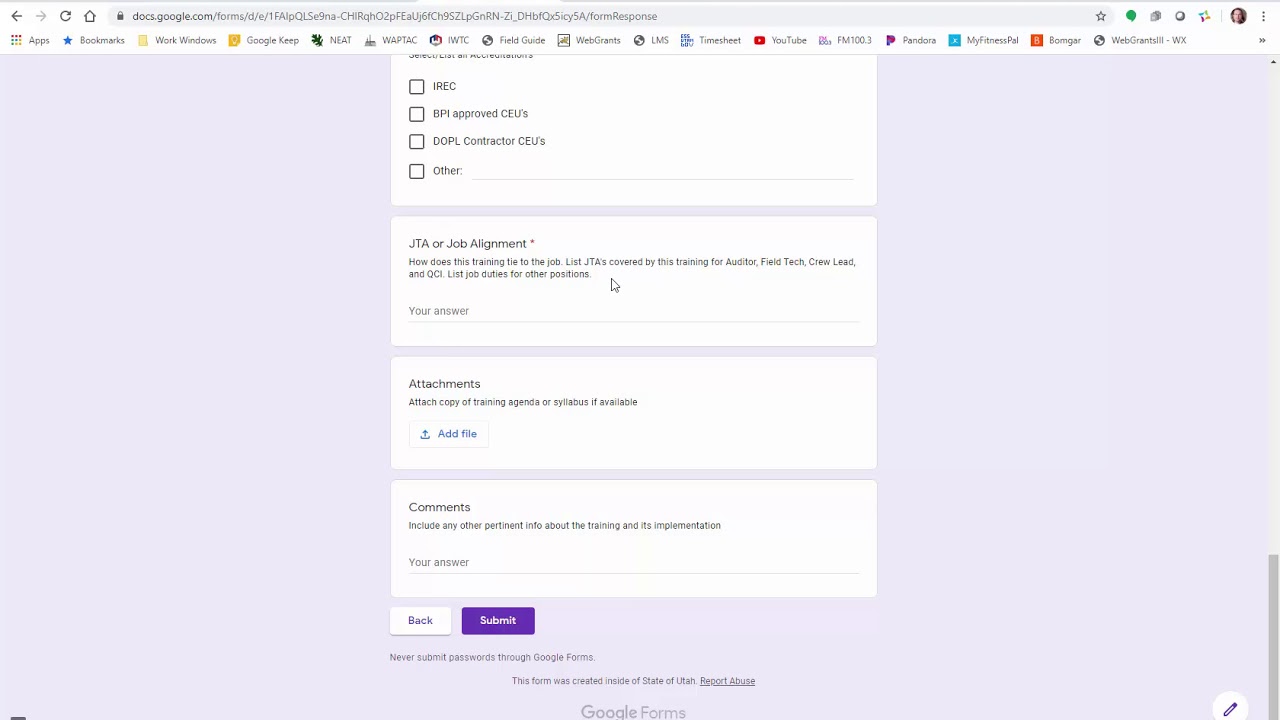The image is a screenshot of a Google Form displayed within the Google Chrome web browser, showcasing various interface elements and details. At the top of the browser, the URL bar displays a web address beginning with "docs.google.com/forms/", followed by an extensive string of characters. The bookmarks toolbar is visible below the URL bar, featuring bookmarked items such as YouTube, MyFitnessPal, Pandora, Work Windows, Google Keep, and several others.

Centered within the browser window is the Google Form, composed of four distinct sections set against an almost imperceptibly light lavender background. The first section appears to be a list of items. The second section, titled "JTA or Job Alignment," is written in gray text. This section prompts users with the question, "How does this training tie to the job? List JTAs covered by this training for author, field tech, crew lead, and QCI. List job duties for other positions." Beneath this prompt is a designated space for responses.

The third section is labeled "Attachments" and encourages users to attach a copy of the training agenda or syllabus if available. The final section, titled "Comments," asks for any other pertinent information about the training and its implementation, offering space for additional input.

At the very bottom of the form are two buttons. The "Submit" button, a purple rectangle with white text, is positioned to the right, while the "Back" button, a white rectangle with gray text, is located to the left. These interactive elements conclude the form, ready for user interaction.